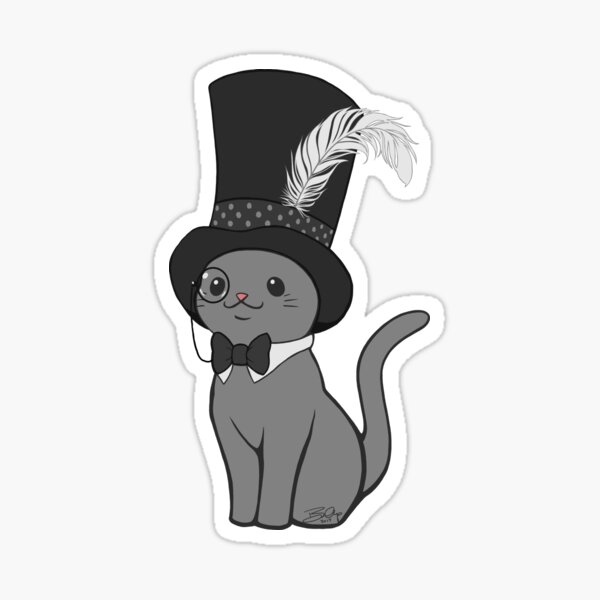This image is a vertically rectangular, monochrome drawing of a charming gray kitten, styled as a cartoon character. The adorable feline is seated, slightly turned to the left, with a visible pink nose, a bright smile, and short whiskers. Both of its eyes are large black circles with small white dots to indicate the pupils. The kitten exudes an air of sophistication, wearing a black bow tie and a small white collar around its neck. Adding to its distinguished look, the kitten sports a black monocle on its left eye (the right eye of the viewer), and a prominent black top hat adorned with a polka dot band and a long white feather curved elegantly toward the back. The background of the image is a faint gray, almost unnoticeable, giving the drawing a subtle contrast. Adding to the impression that this might be a sticker, there's a lighter blue outline forming a border around the kitten, set against an off-white background. There appears to be a faint signature on the back leg of the kitten, though it is too small to decipher.